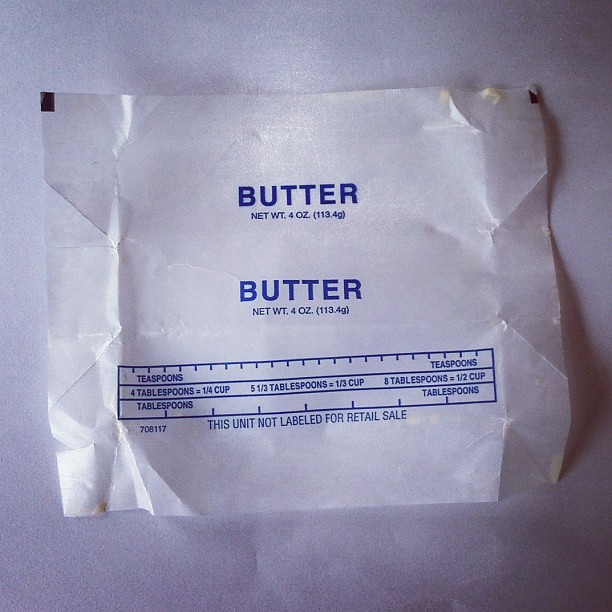The image depicts an unfolded, opaque white butter wrapper lying flat on a white surface, likely a countertop or table. This wrapper originally encased a 4-ounce (113.4 grams) stick of butter, with traces of butter still visible on it. The wrapper, clearly marked with "Net weight: 4 ounces" and its conversion to grams, includes standard measurement markings for easy portioning. These markings detail that eight tablespoons equals half a cup, five and a third tablespoons is a third of a cup, and four tablespoons is a quarter cup. Additionally, there are individual tablespoon indicators. The wrapper also notes that the unit is not labeled for retail sale, indicating it came from a larger multi-pack.